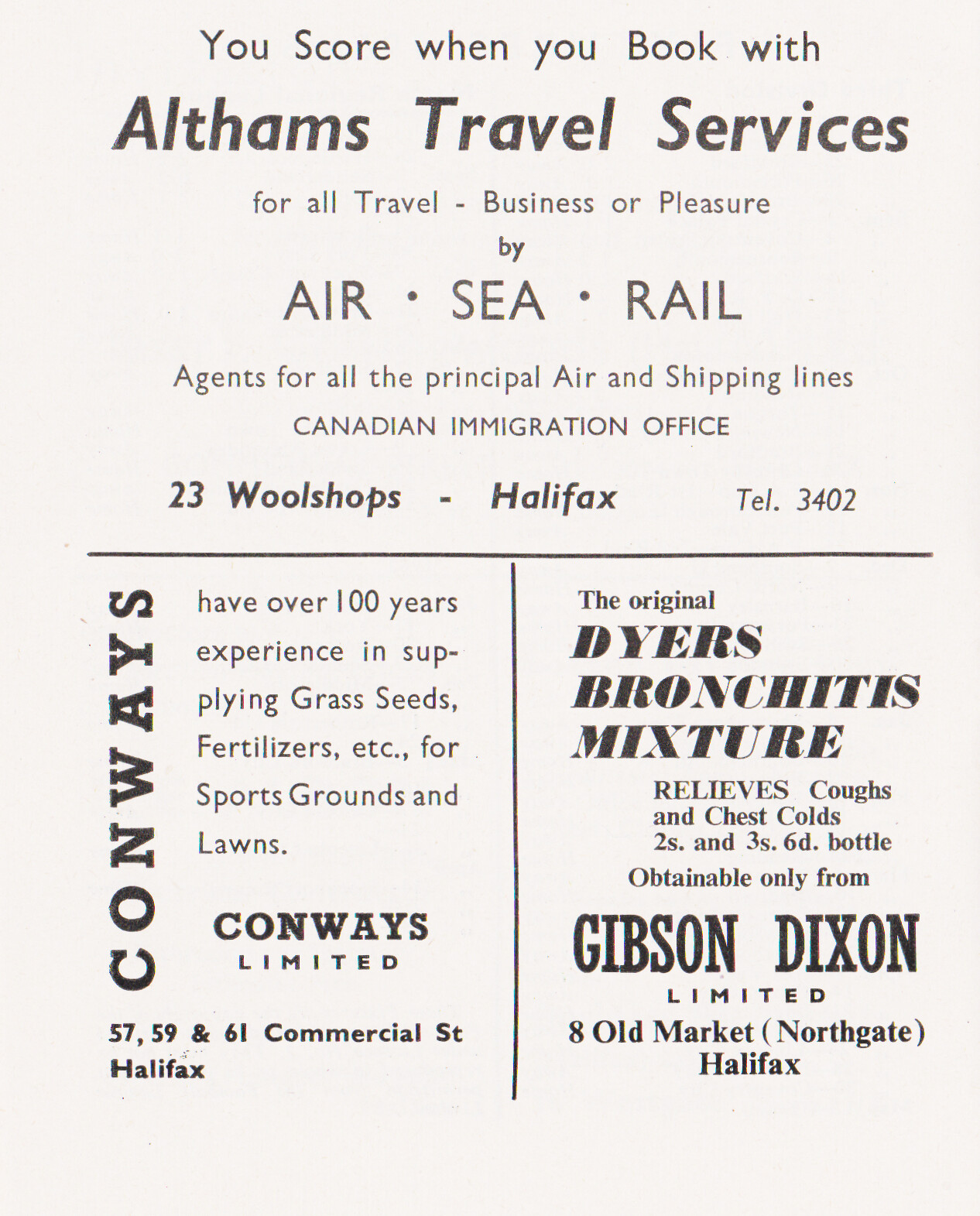This image appears to be a page, likely from a pamphlet or magazine, featuring three distinct advertisements set against a white background with black text. The top half of the page prominently displays an ad for Altham's Travel Services, proclaiming "You score when you book with Altham's Travel Services for all travel, business, or pleasure by air, sea, and rail." The ad highlights Altham's as agents for all principal air and shipping lines and includes a mention of the Canadian Immigration Office. The address provided is "23 Woolshops, Halifax," with a telephone number of "3402."

Below this, the page is divided into two separate framed advertisements. The frame on the left promotes Conway's, stating that they have over 100 years of experience in supplying grass seeds, fertilizers, and other products for sports grounds and lawns. The address listed for Conway's Limited is "57, 59, and 69 Commercial Street, Halifax."

The frame on the right advertises "the original Dyer's Bronchitis Mixture," which is noted to relieve coughs and chest colds. It is available in bottles priced at "2S and 3S 6D," and can be obtained exclusively from Gibson-Dixon Limited, located at "8 Old Market, Northgate, Halifax."

Overall, the structured layout and cohesive design suggest this is a carefully arranged page meant to inform readers of various local services and products.